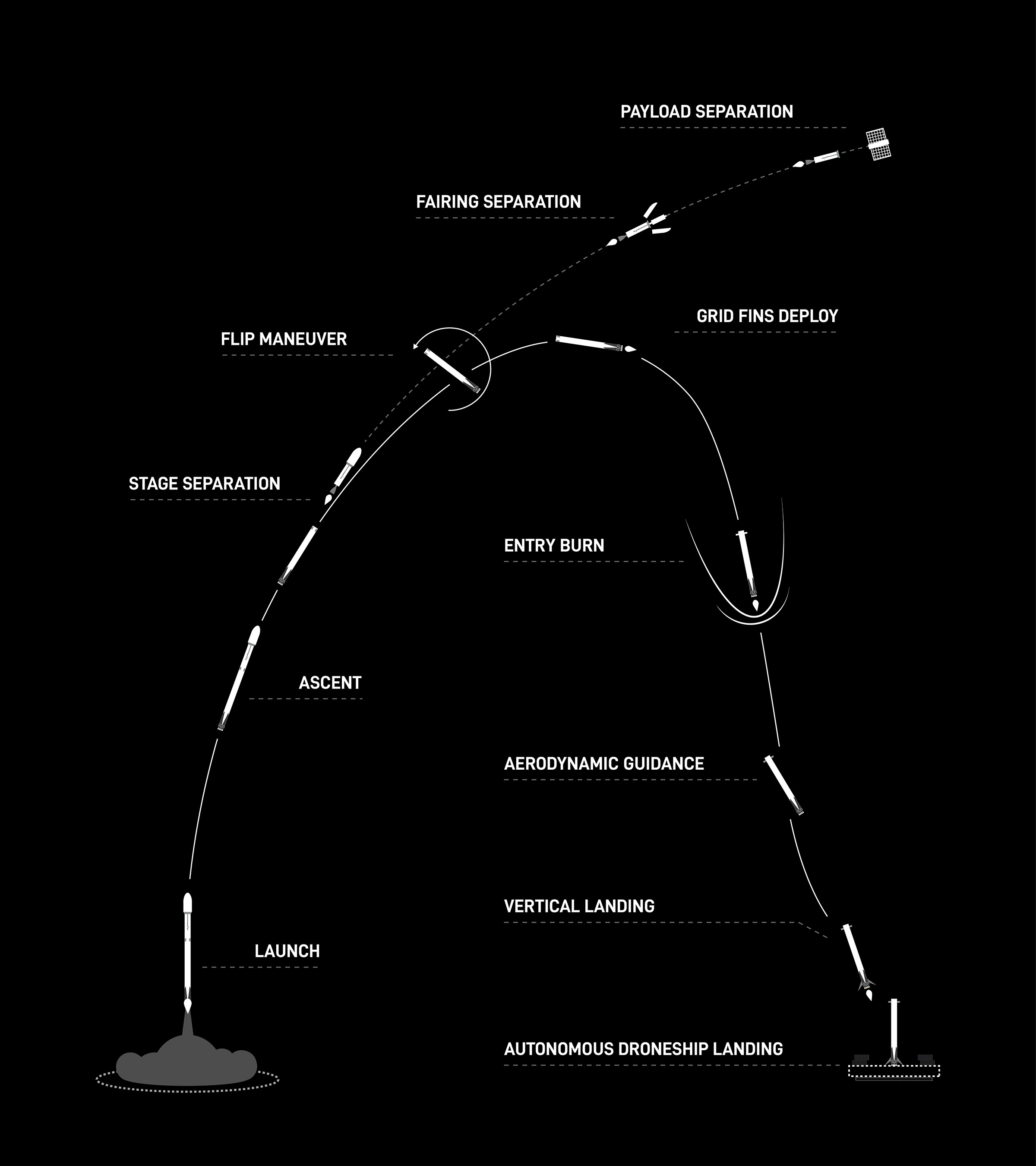The image is a highly detailed, black and white diagram depicting the various stages of a rocket's launch and landing sequence, set against a completely black background. Starting from the lower left, the rocket is illustrated with the label "launch" beside it and a plume of gray smoke underneath. The trajectory curves upward to the right with the labeled stages: "ascent," "stage separation" where the rocket separates into parts, and "flip maneuver." Higher up in the arc, the steps "fairing separation" and "payload separation" are depicted, showing the rocket's different components breaking away. 

At the apex of the arc, the diagram splits into two paths. One path continues to rise, while the other shows the rocket in descent, labelled with "grid fins deploy," "entry burn," "aerodynamic guidance," "vertical landing," and "autonomous drone ship landing" as it curves back to earth. This detailed imagery effectively illustrates the complete launch-to-landing process of the spacecraft, highlighting both its ascent and its capability to return and land upright.